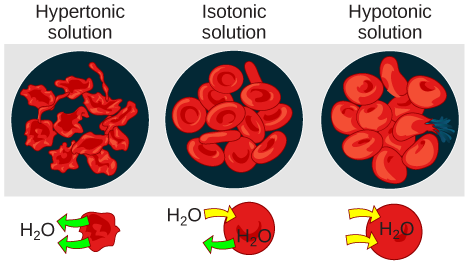The image is a digitally illustrated diagram divided into three sections within a light gray rectangle over a white background. Each section has a black circular background containing objects resembling red blood cells, and each section is labeled at the top. The left circle, labeled "hypertonic solution," features red blood cells with a wobbly appearance. Below this circle is an illustration of one of these cells with two green arrows pointing towards it, signifying the movement of water (H2O) into the cell. The middle circle, labeled "isotonic solution," depicts normal-looking red blood cells. Underneath it, H2O arrows are depicted: a yellow arrow moving into the cell and a green arrow moving out, representing equilibrium. The right circle, labeled "hypotonic solution," shows red blood cells that appear overly full, with one looking like it is bursting. Below this is an illustration of a cell with two yellow arrows pointing towards it, again indicating water movement. Each section effectively visualizes how red blood cells respond to different types of solutions in terms of water (H2O) movement.